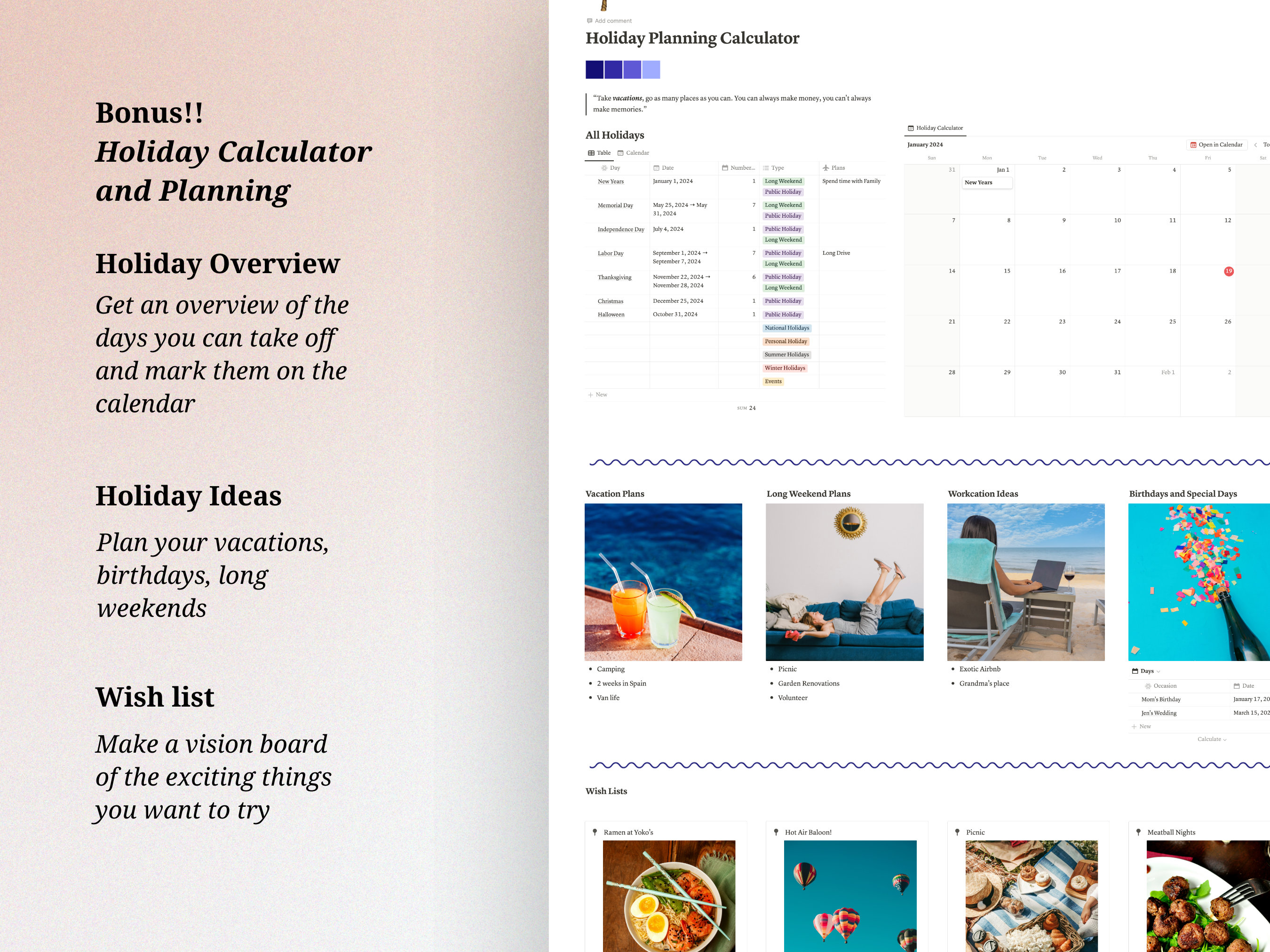This image is a detailed screenshot of a web page featuring several sections related to holiday planning and personal organization. 

**Left Side:**
- **Background Color**: Dark pink.
- **Content**:
  - **"Bonus!!"** (Bold Black Text)
  - **"Holiday Calendar"** (Bold Black Text, New Line)
  - **"In Planning"** (Bold Black Text, New Line)
  - **"Holiday Overview"** (Bold Black Text, New Line)
  - **Description**:
    - Get an overview of the days you can take off and mark them on the calendar.
  - **"Happy Ideas"** (Bold Black Text)
  - **Description**:
    - Plan your vacations, birthdays, long weekends.
  - **"Wish List"** (Bold Black Text)
  - **Description**:
    - Make a vision board of the exciting things you want to try.

**Right Side:**
- **Main Feature**: A detailed schedule next to a white calendar with the date 18th circled in red.
- **Title**: "Holiday Planning Calendar" (Bold Black Text, Top Left)
- **Color Squares**: 
  - **Purpose**: Denote different types of activities.
  - **Colors**: 
    - Dark Purple
    - Lighter Dark Purple
    - Mid Purple
    - Blue-ish Purple
- **Sections**:
  - **Holidays** (Black Text, Left Hand Side)
  - **Tags**: Color-coded with green, purple, orange, and red.

**Images and Descriptions**:
1. **Two Glasses**: One with orange liquid, one with yellow liquid, against a light brown pool edge.
2. **Female on Sofa**: Dressed in all gray, laying on a dark blue sofa.
3. **Female with Laptop**: Sitting in a teal blue chair with a backdrop of a blue sky, white clouds, and a tan beach.
4. **Confetti**: Various colors including purple, hot pink, pink, green, yellow, and red.
5. **Close-Up Ramen**: Tan noodles, two white eggs with yellow yolks, light blue chopsticks with black designs, and tomatoes.
6. **Hot Air Balloons**:
    - Multiple colors including blue, red, white, yellow, dark blue.
7. **Donuts**: White, brown, and powdered, on a picnic blanket with white, cyan blue, and dark blue stripes.
8. **Meatballs**: Brown with slight burning on greens, fork inside one of them.

This comprehensive view combines visual elements and text to create an interactive and vibrant holiday planning experience.